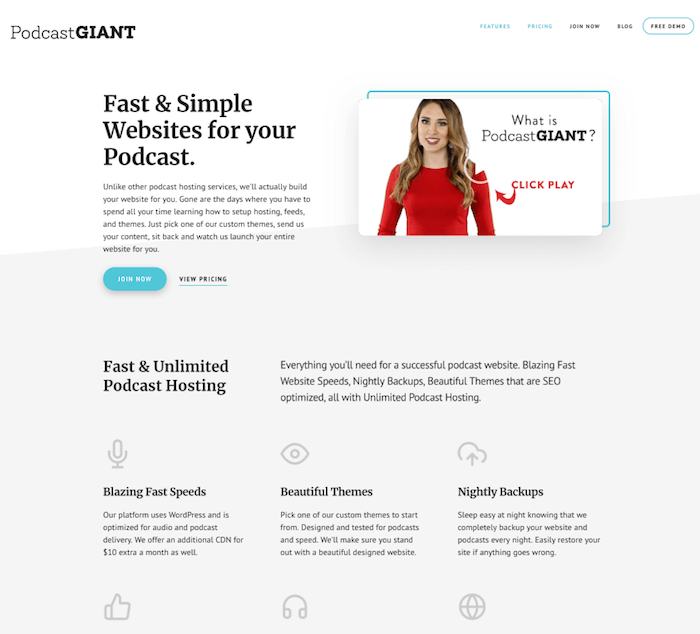The image showcases a podcasting website with a streamlined interface. In the top left corner, the website name "Podcast Giant" is prominently displayed, with "Podcast" in regular font and "Giant" in bold font to the right. The top right section features five categories; the first two are in light blue, while the last three are in black with the final one outlined in light blue.

A headline below reads "Fast and Simple Websites for Your Podcasts" followed by a brief paragraph and an option in light blue text labeled "View Pricing" in black. Adjacent to this is an image of a smiling woman wearing a red shirt, with accompanying text "What is Podcast Giant?" Below this, in red text, the phrase "Click Play" is prominently displayed.

Further down, a description emphasizes "Fast and unlimited podcast hosting, everything you'll need for a successful podcast website." It highlights key features such as "Blazing fast website speeds, nightly backups, and beautiful themes that are SEO optimized," all supported by unlimited podcast hosting.

The section following this has three icons: a microphone labeled "Blazing Fast Speeds," an eye labeled "Beautiful Themes," and another set of icons with descriptions: a thumbs-up, headphones, and a globe. Each icon is accompanied by detailed information in small text. The entire bottom half of the site features a light gray background for a cohesive look.